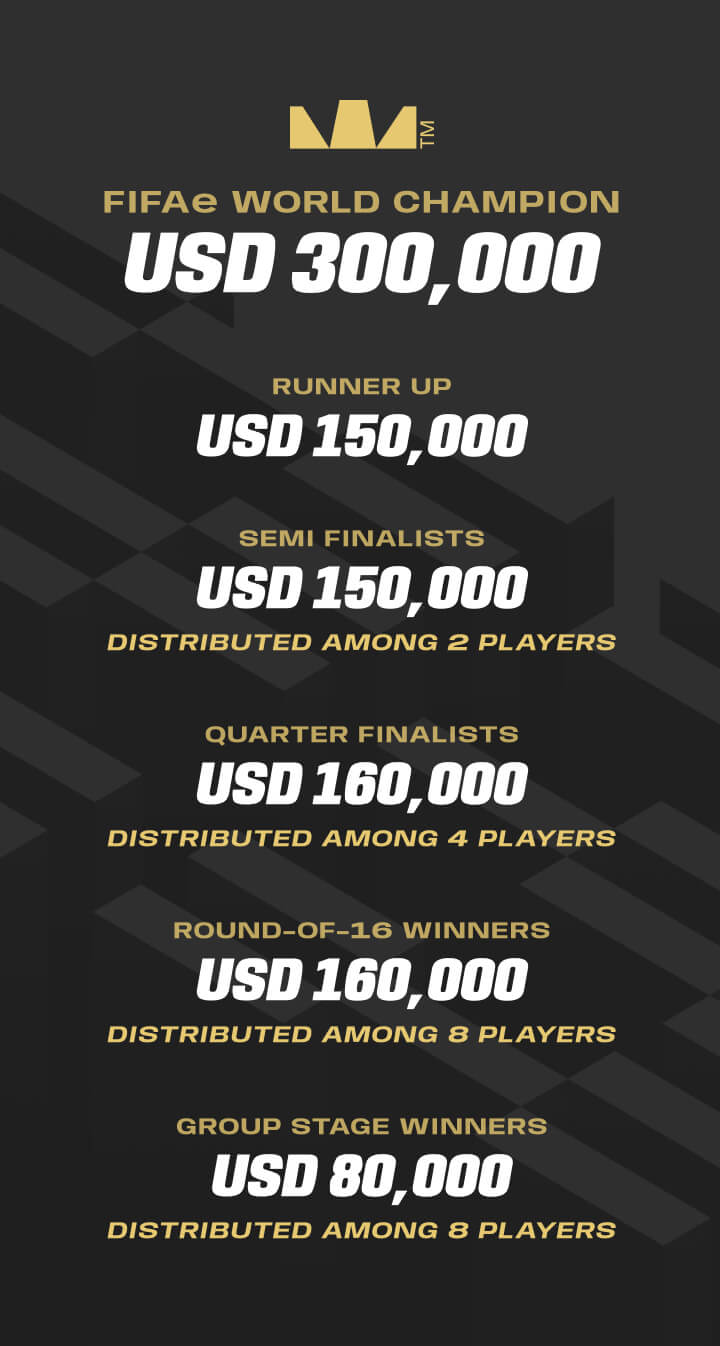The image is a banner with a black and gray 3D block texture background that primarily contains text. At the top of the banner, there is a stylized gold crown logo with a trademark symbol. Below the logo, in prominent letters, it reads "F.I.F.A.E World Champion." The prize amounts are listed in white text: "World Champion USD 300,000," "Runner-Up USD 150,000," "Semi-Finalists USD 150,000, distributed among two players," "Quarter-Finalists USD 160,000, distributed among four players," "Round of 16 Winners USD 160,000, distributed among eight players," and "Group Stage Winners USD 80,000, distributed among eight players." The banner does not contain any photographic elements or images of people; it is solely text and graphic design.